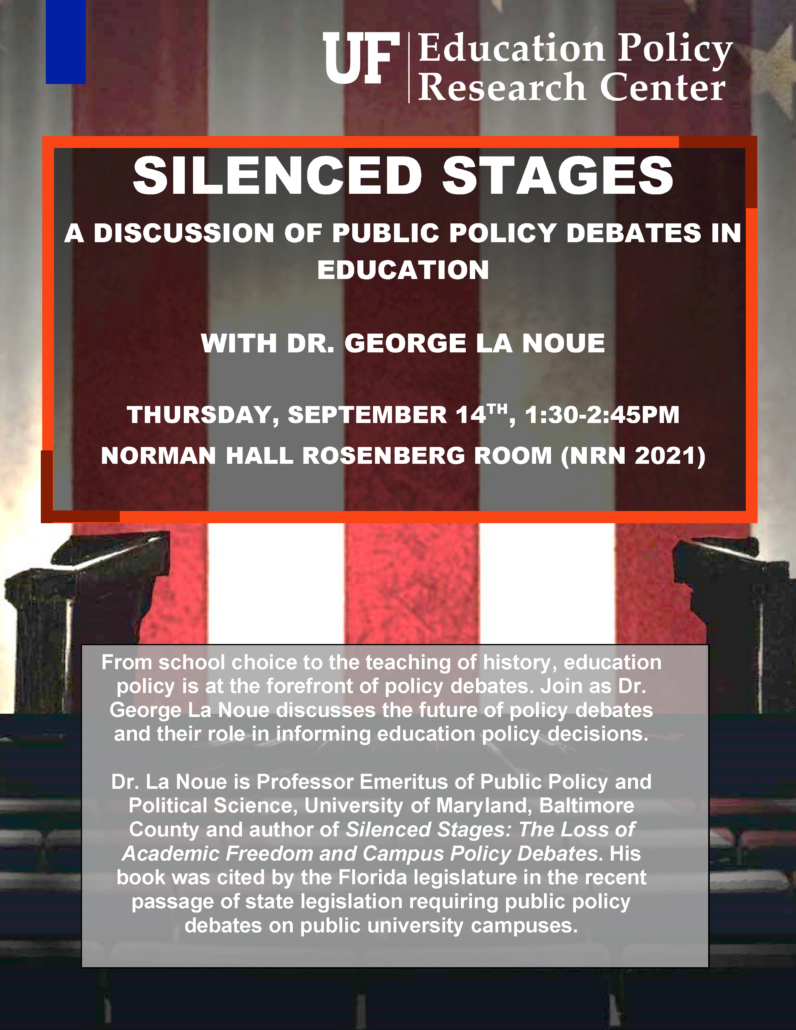The image is a detailed flyer for an event hosted by the UF Education Policy Research Center. At the top, the title "UF Education Policy Research Center" is displayed in white text against a background featuring vertical red and white stripes, resembling the American flag, with a blue rectangle in the upper left corner and a star in the upper right corner. Below this, there is a red-bordered gray rectangle with the bolded title "SILENCED STAGES" in white capital letters. Further down, smaller text outlines the event specifics: "Discussion of Public Policy Debates in Education with Dr. George Lanoun, Thursday, September 14th, 1.30 to 2.45pm, Norman Hall, Rosenberg Room, NRN 2021." The bottom section of the flyer, set against a semi-transparent gray background, provides more context: "From School Choice to the Teaching of History, Education Policy is at the Forefront of Policy Debates. Join as Dr. George Lanoun discusses the future of policy debates and their role in informing education policy decisions." Additionally, Dr. Lanoun is described as a Professor Emeritus of Public Policy and Political Science at the University of Maryland Baltimore County and the author of "Silenced Stages: The Loss of Academic Freedom and Campus Policy Debates." The background image at the bottom of the flyer appears to depict an auditorium or stage area, symbolizing the setting for the discussed debates.